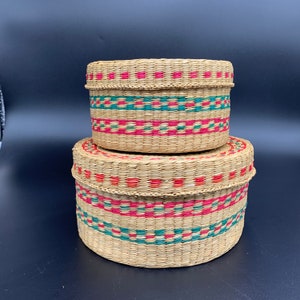This is an image of two identical woven round baskets made of pale straw with intricate pink and blue stripes. The larger basket sits at the bottom, while the smaller one is placed on top of it. Both baskets have lids with braided edges that move on and off. The lids feature pink sections woven into the design, adding a decorative touch. The background is a variegated navy blue with streaks of grayish blue, making the baskets stand out vividly. The texture of the baskets is clearly visible, allowing one to appreciate the handmade quality, which gives them a South American or Native American aesthetic. Overall, the image conveys a sense of vibrant craftsmanship and cultural artistry.